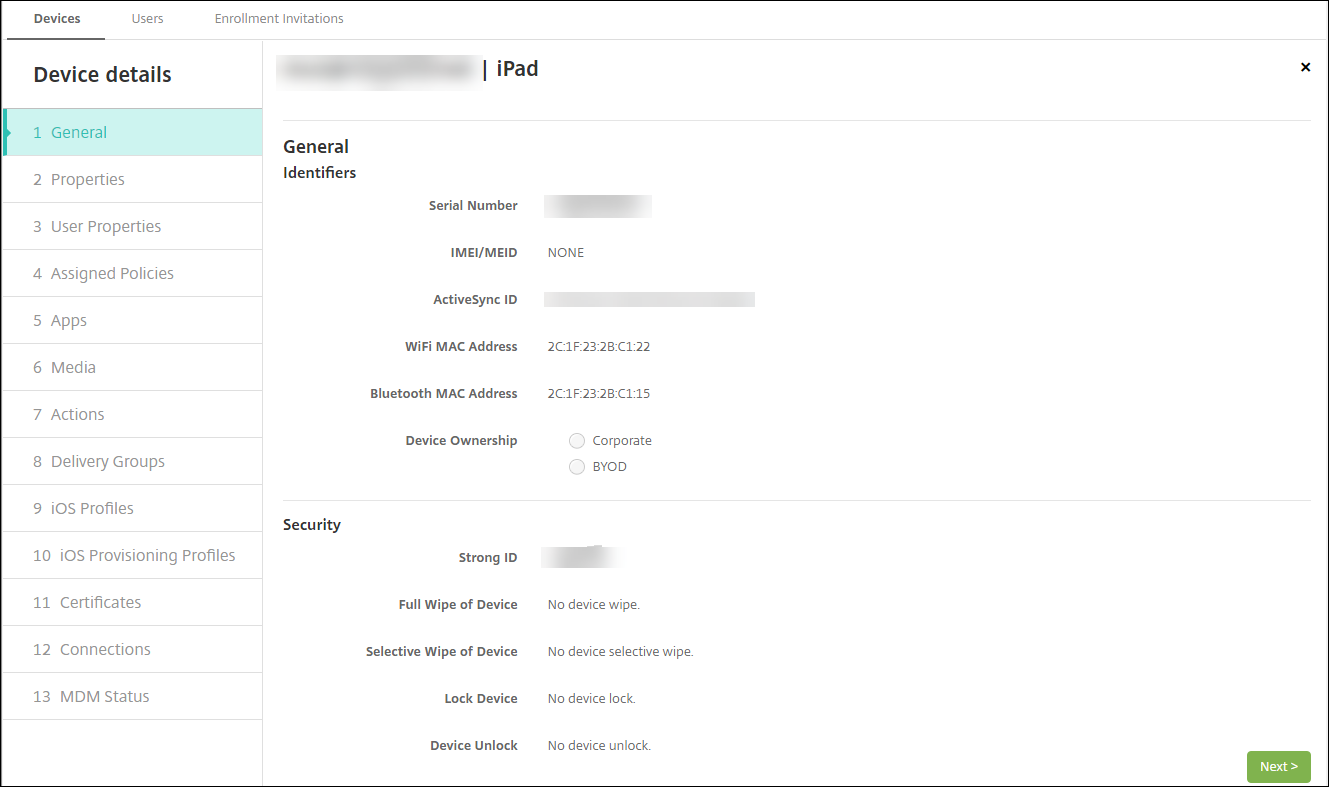This screenshot appears to be taken from an iPad in landscape orientation. The interface can be divided into a few main sections. At the top, three tabs are visible: "Devices," "Users," and "Enrollment Invitations." On the left side of the screen, there is a detailed navigation menu that lists 13 different categories: General, Properties, User Properties, Assigned Policies, Apps, Media, Actions, Delivery Groups, iOS Profiles, iOS Provisioning Profiles, Certificates, Connections, and MDM Status.

The highlighted category on the left is "General," which displays detailed information on the right side of the screen. In this section, several data points are either grayed out or blurred to protect sensitive information. These include the serial number, ActiveSync ID, and a strong ID under the security settings. The IMEI or MEID field shows "None."

Additional technical details are provided, such as the Wi-Fi MAC address and the Bluetooth MAC address. The ownership of the device is not specified, as neither "Corporate" nor "BYOD" (Bring Your Own Device) is selected.

Towards the bottom of the screen, under the "Security" section, several options are visible but none are currently selected. These options include "Full Wipe of Device," "No Device Wipe," "Selective Wipe of Device," "Lock Device," and "Device Unlock."

This detailed view allows for comprehensive management and oversight of the iPad, though all sensitive and identifying information has been appropriately obscured for privacy reasons.